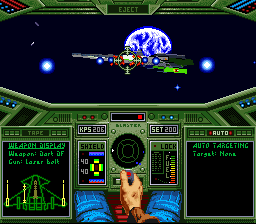This screenshot from a vintage-style video game, reminiscent of those from over two decades ago, offers an immersive point-of-view experience. The scene is viewed from the cockpit of a spaceship navigating outer space. Inside the cockpit, visible in detailed retro graphics, a character dressed in blue jeans and a long-sleeved shirt grips a joystick with a red button on top. Surrounding the character are various control panels and screens emitting green and yellow hues, displaying commands like "shield lock" and "auto-targeting." Through the spaceship's windshield, the vastness of space unfolds with a starry black background. 

Directly ahead, another spaceship appears, locked in the player’s targeting system, indicated by a green circle and arrows. Beyond this, the planet Earth is visible in the distance, a striking blue orb adorned with white clouds. This setup suggests a mission or combat scenario, possibly aimed at protecting Earth from threats. The detailed point-of-view format draws the player into the high-stakes space adventure, blending nostalgic elements with an engaging gameplay experience.